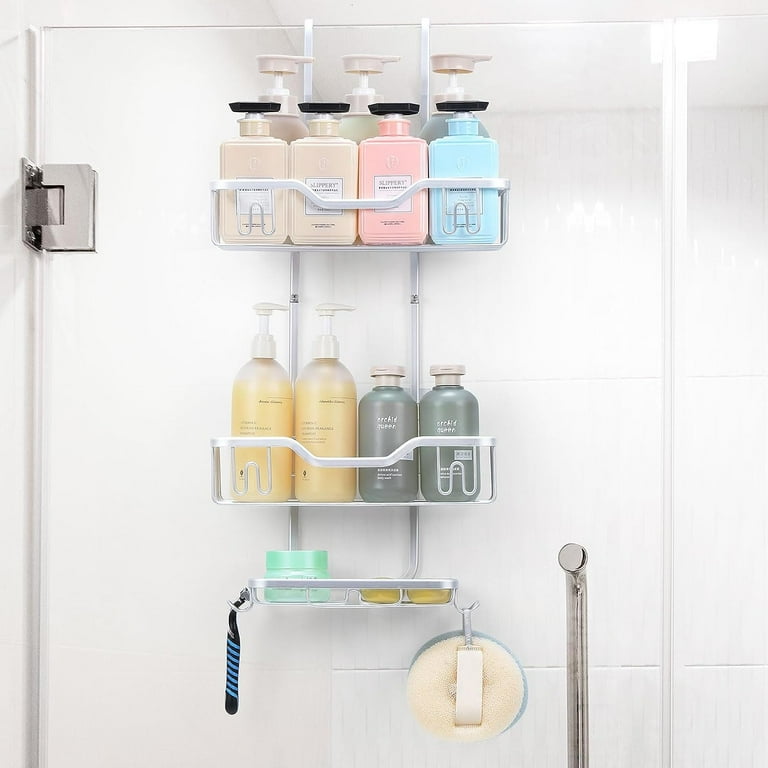This photograph, taken in portrait view, offers a detailed, up-close look at the inside of a shower, focusing on the glass door and the hanging caddy of toiletries. The shower door is clear glass with a silver handle positioned towards the bottom right corner and silver bolts on the left-hand side. In the middle of the door, a three-tier caddy is suspended, organizing an array of bottles and personal care items.

The top tier of the caddy features seven bottles: three tall pump bottles in the back and four shorter squeeze bottles in the front. These bottles come in various shades including tan, pink, and blue, with most being tan except for the two shorter bottles on the right—one baby blue and one baby pink.

The second tier holds four bottles: two taller pump bottles on the left filled with a gold or yellow liquid, and two shorter, dark gray or dark green bottles on the right.

On the bottom tier, there are two bars of soap and a small cylindrical container, possibly for lip balm. A black and blue striped razor hangs on the left side of this tier, while a loofah, colored tan and blue, dangles on the right. The door frame is outlined by a white seam on the right and a stainless steel hinge on the left, adding to the structure and detail of this carefully organized shower space.